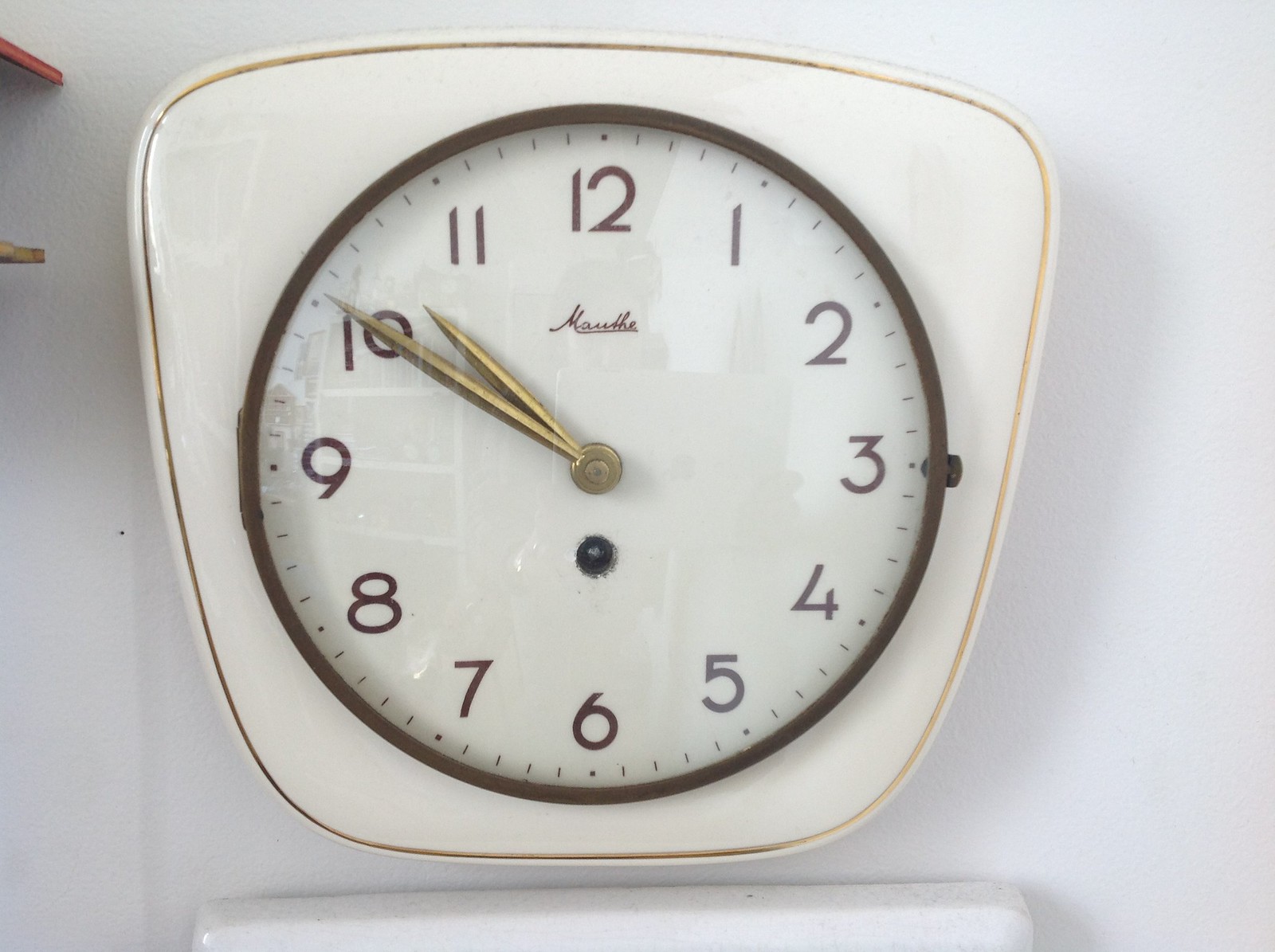This photograph showcases a uniquely designed square clock with a retro flair. The main body of the clock is white, encased by a thin gold trim that outlines its squared shape. At the center of the clock is a dark brown or black circular accent, which complements the white clock face. The clock features gold hands that stand out elegantly against the background. Each numeral on the clock is rendered in a dark brown shade, paired with a series of dark brown dash marks encircling the numbers, adding to the vintage aesthetic. Below the clock, a partial view of another white, square-shaped object is visible, though its exact purpose is indeterminate. Additionally, the image captures a glimpse of shelving on one side, featuring a red piece and a section made from blonde wood. The white wall against which the clock is mounted displays the shadow of the clock, enhancing the overall composition of the photograph.